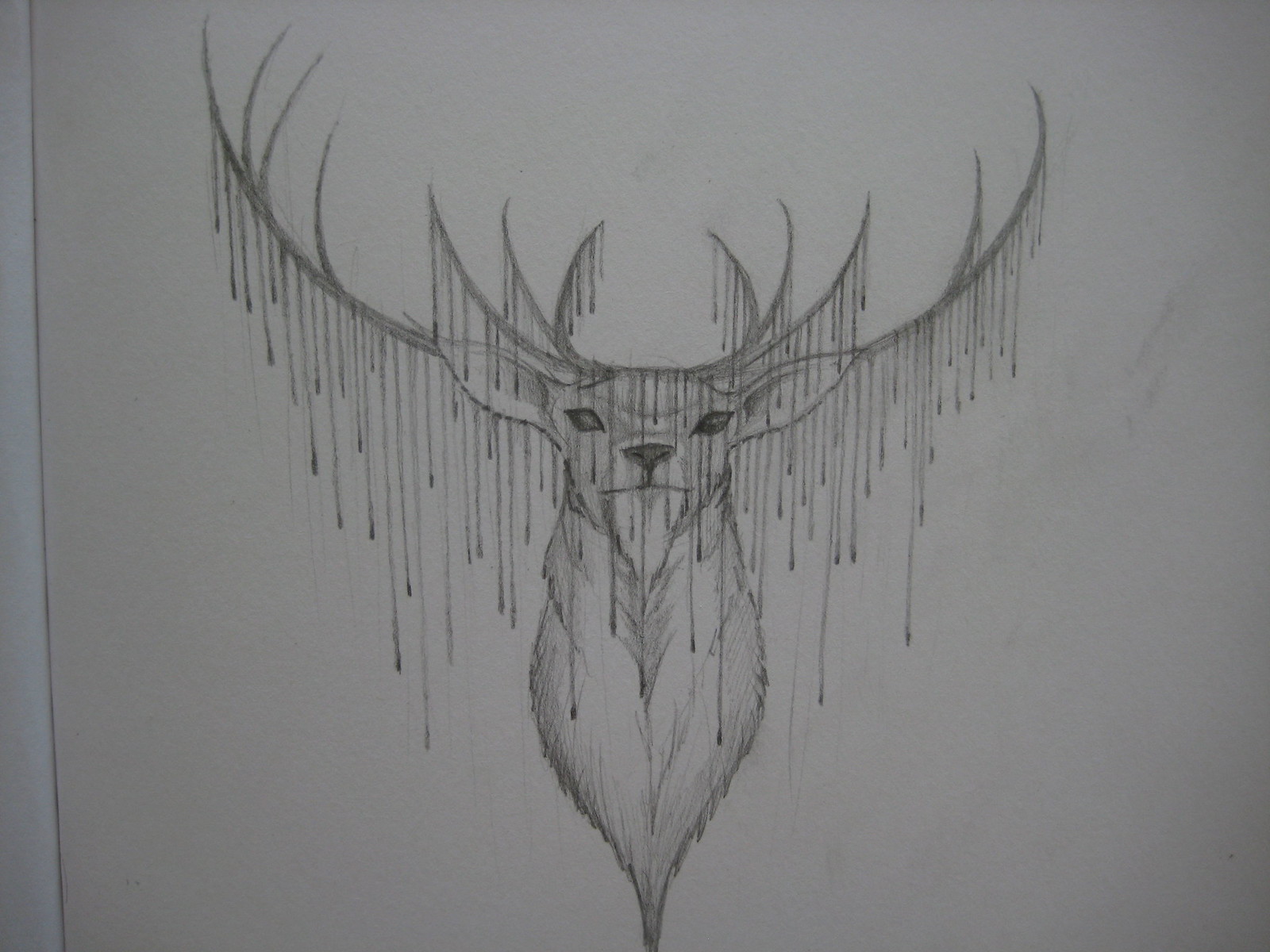This intricately detailed pencil drawing features the head of a majestic deer, prominently facing forward. The deer boasts an impressive set of antlers with 12 points adorned with what appears to be delicate drops or tinsel hanging from each horn. Though the artist has focused primarily on the neck and head, the sketch captures the lifelike texture of the deer's fur with meticulous strokes, giving it a realistic and tactile quality. The white backdrop of the paper adds a stark contrast, highlighting the precision and depth of the pencil work. The deer’s body is not visible, ending just below the neck, allowing the viewer’s gaze to remain fixed on the elaborate antlers and expressive, lifelike face.